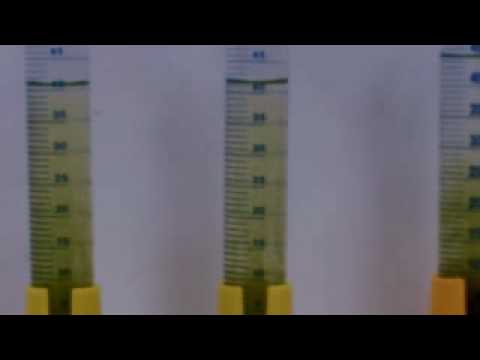The image appears to be a low-resolution screenshot from a video, depicting three clear plastic vials filled with a gradient liquid that transitions from a darker hue at the bottom to a clearer appearance at the top. Each vial has black numbers and measurement lines along the side, making it easy to read the liquid levels. The vials are mostly full, with the one on the far right being slightly fuller than the other two. The liquid inside the vials seems to have a yellow-green tint, becoming darker near the bottom, suggesting it might be contaminated water. The vials are placed in yellow plastic holders that clasp around their bases, leaving an open space between them. The setup is positioned against a white background, which casts shadows from the vials, and there are black bars at the top and bottom of the image. Noticeable compression artifacts affect the image quality.